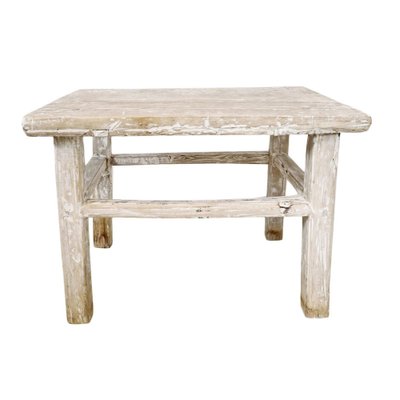This image depicts a photograph of an aged, weathered wooden table. The table is relatively small, akin to the size of a nightstand, standing about three feet tall. Its structure features a rectangular shape, with an estimated width of three feet and a length of four feet, offering a slightly greater lengthwise dimension. The table comprises four legs, each connected by narrow horizontal beams, which enhance its stability.

The wood of the table is notably worn and weathered, exhibiting a light color palette that shifts between light gray and very light brown hues. There is evidence of a sheer white paint or similar substance applied unevenly across its surface, giving the table a textured, white-accented appearance where the natural wood grain is visible, especially on the back horizontal beam. The bottom portions of the legs are distinctly darker, transitioning to a dark brown shade that suggests dirt and age. The table, with its rustic charm and well-worn character, conveys a sense of history and endurance.